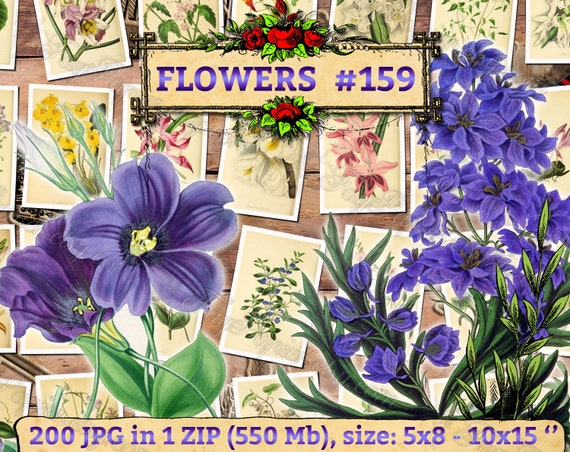The rectangular image, approximately four inches wide and three inches high, features a collage of floral illustrations against a background of horizontal brown wood slats. Central to the image are rows of small cards framed with white borders and a beige background, each depicting colorful flowers in hues of yellow, pink, and white. Overlaying these cards, in the lower left corner, is a detailed illustration of a large five-petaled purple flower with yellow stamens and green leaves. On the right, blossoms resembling lavender grow in bushels with alternating patterns along green stems. Dominating the top of the image, a beige rectangular banner with red roses and green leaves features purple gradient text that reads "Flowers Number 159." At the bottom of the image, another beige banner with a black outline contains additional purple text: "200 JPG in one zip, 550 MB, size 5x8 - 10x15." The vivid combination of floral art and detailed text hints at an advertisement for a digital collection of flower images.